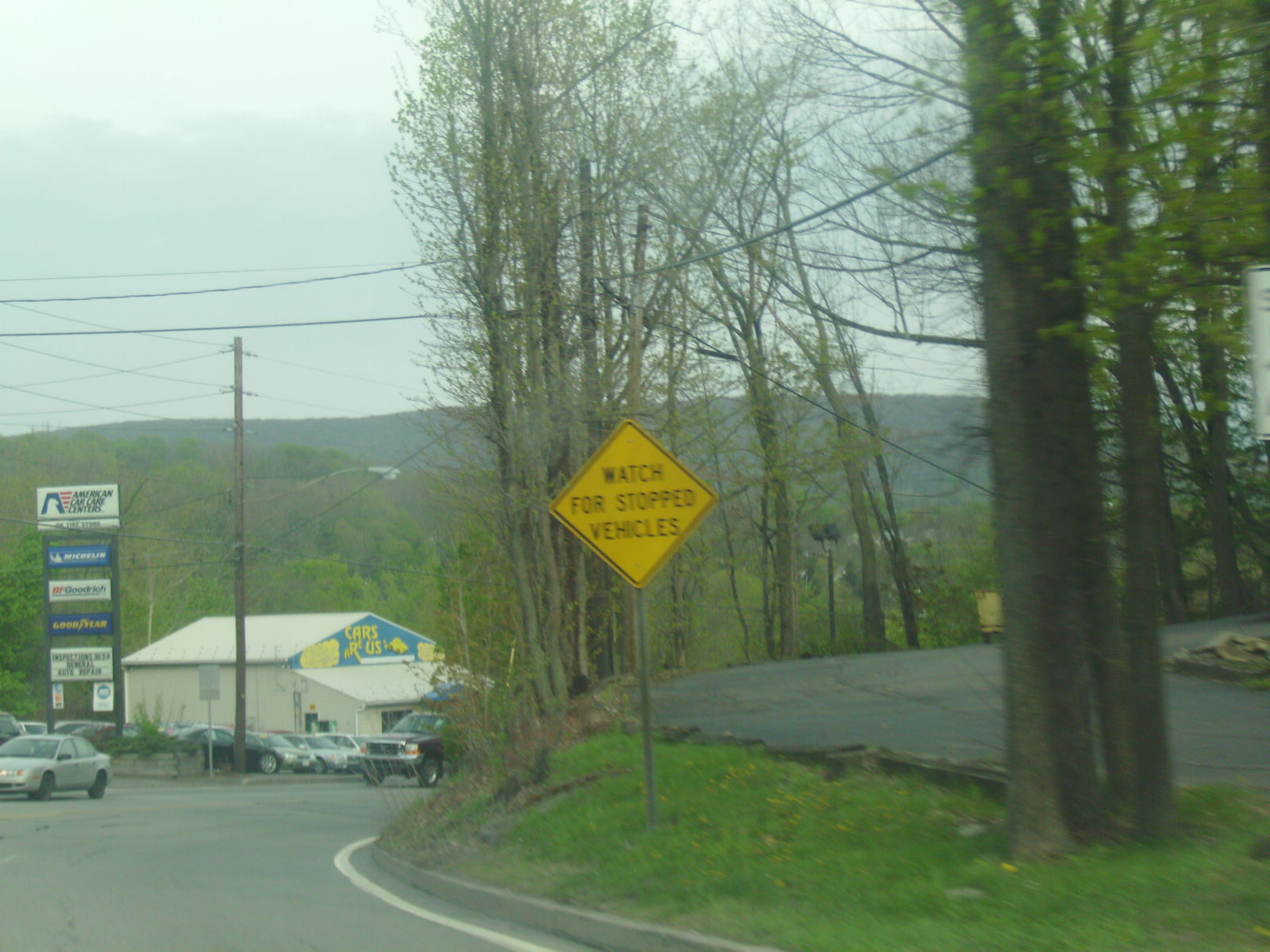This photograph, taken on a hazy day with uncertainty whether due to cloudy weather or air pollution, depicts a tranquil yet dynamic scene. The sky transitions from a very pale blue at the top to a more subdued gray, indicative of heavy cloud cover. On the right-hand side, a slight hill rises above the main road to the left, featuring a curving paved area whose function—perhaps a driveway—remains unclear. Early spring is evidenced by the trees, just beginning to bud, mingled with an evergreen. Below, green grass lushly carpets the ground.

To the left, the main road snakes around a white, unpretentious building labeled "Cars Plus." This straightforward structure is accompanied by telephone poles strung with wires and a cautionary traffic sign. The sign, mounted on a gray metal post and set against a yellow background, warns drivers to "watch for stopped vehicles." Its positioning alerts motorists about the visibility challenges posed by the road’s bend near the car lot.